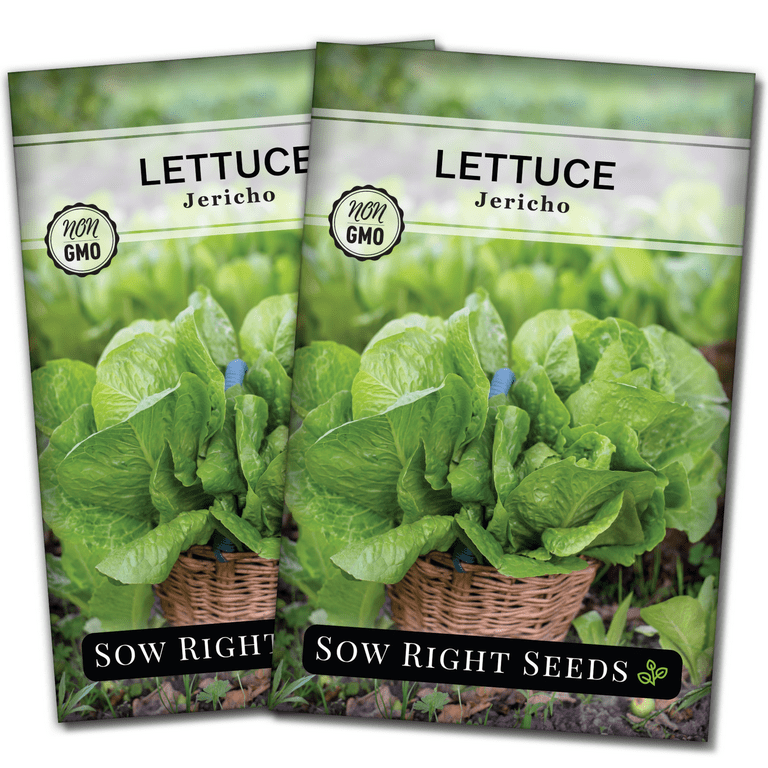This image features two identical seed packets displayed side by side, with the packet on the right slightly overlapping the one on the left. Each packet has a bright and vibrant design, showcasing a lush head of green lettuce emerging from a brown wicker basket. At the top of the packet, there's about an inch of out-of-focus green plants, followed by a thin gray border with a green streak. Below this is a thick gray banner stretching across the packet, where the word "Lettuce" is prominently printed in large black letters, with "Jericho" written in smaller lettering underneath.

On the bottom left of the gray banner, a gray circle with a black border houses the words "NON-GMO" in black letters. Below the thick gray banner, the image resumes with slightly out-of-focus greenery and soil, depicting a natural, farm-like setting, complete with scattered rocks and dead leaves.

At the very bottom of the packet, a black banner features the text "Sow Right Seeds" in white letters, with a green illustration of a plant with three leaves beside the word "Seeds." The overall presentation effectively emphasizes the product's organic and vibrant nature, encouraging a lush green harvest.